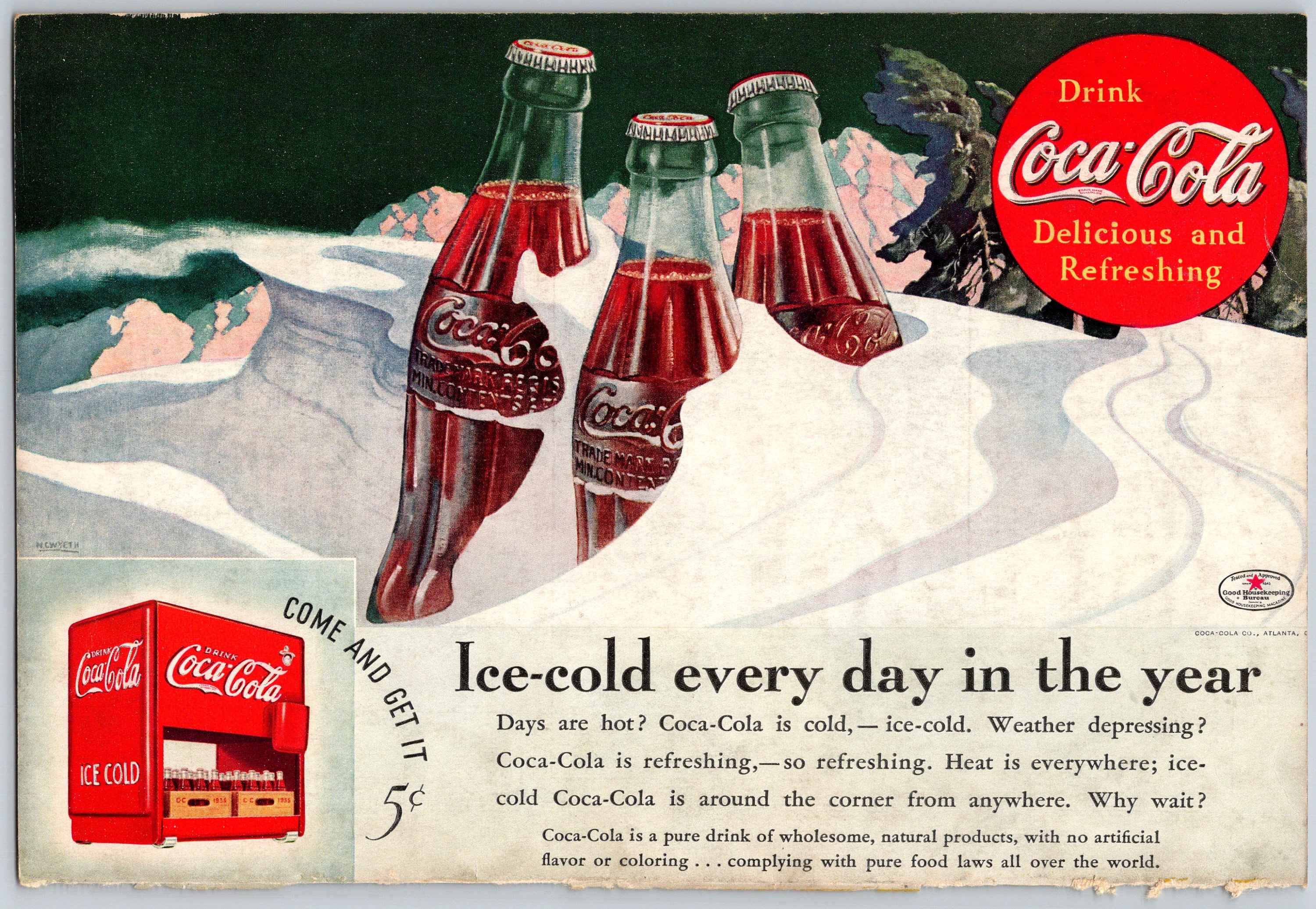This is a vintage Coca-Cola advertisement set against a wintery backdrop of snow-covered mountains, trees, and a dark night sky with snow drifting in the background. At the center of the image, three classic glass Coca-Cola bottles are buried in snow, their necks and iconic white logos clearly visible above the snowline, capped with distinct reddish-white caps. The dark brown liquid inside the bottles glistens, hinting at their refreshing coldness. In the top right corner, a bold red circle contains the slogan "Drink Coca-Cola: Delicious and Refreshing" in a yellowish font, highlighting the timeless appeal of the beverage. At the bottom left, an old-fashioned red ice cooler adorned with the Coca-Cola logo is shown, with crates of Coca-Cola bottles neatly stored underneath. The ad also emphasizes its affordability and year-round refreshment with text that reads "Come and get it - Five cents" and "Ice Cold Every Day in the Year." Additionally, nostalgic phrases reinforce the beverage's purity and natural ingredients, reminiscing about its compliance with pure food laws worldwide and its wholesome, artificial-free composition, painting a picture of Coca-Cola as the ultimate refreshment in any weather.